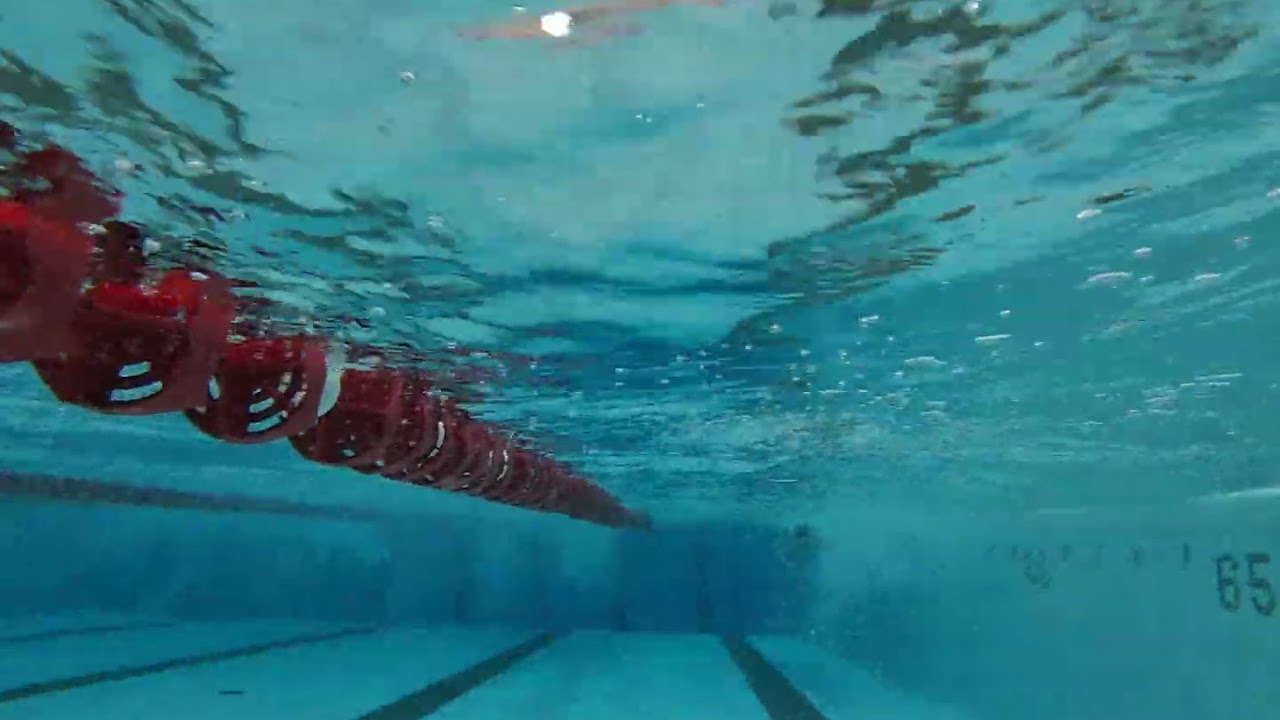This underwater photograph captures the serene environment of a swimming pool. Taken from a submerged perspective, the image offers a unique view of the water's surface overhead, dotted with numerous bubbles and ripples. The water is a light blue, lending the whole scene a crisp, clear quality. Down the length of the pool, you can see black lane lines extending toward the far wall, guiding your gaze forward. On the left side, a rust-colored lane divider composed of identical circular floats lines the pool, floating and separating the lanes. To the right, the pool's wall is marked with the number "65." Both the tiles on the floor and the walls create a vivid, structured layout. The overall composition, with its blend of floating bubbles, lane dividers, and clear visual depth, transports you directly into the quiet, introspective underwater world of the pool.